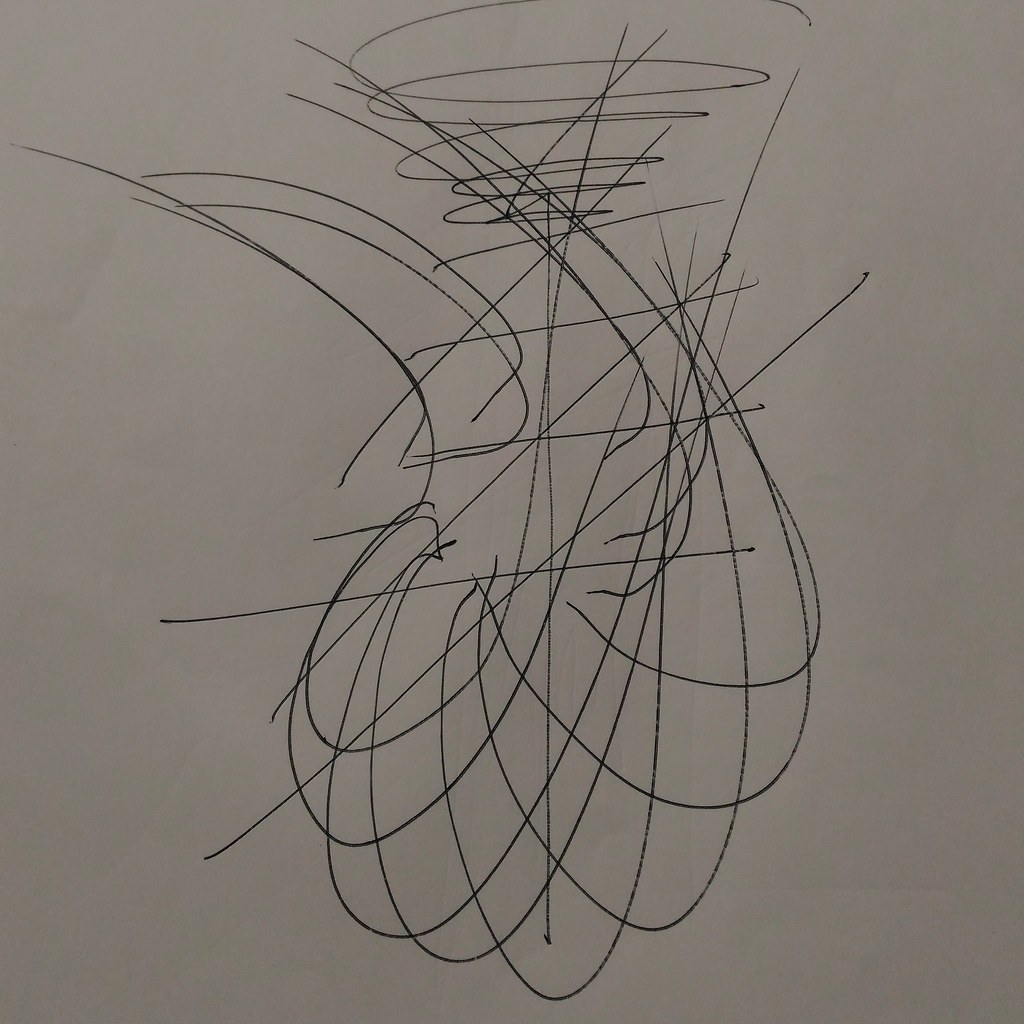This image features an intricate array of black ink scribbles on a white piece of paper, blurring the lines between casual doodling and abstract art. Dominating the composition is a central vertical line intersected by four perpendicular horizontal lines of varying lengths. The lowest horizontal line stretches the longest, while the two middle lines are of similar length and shorter than the bottom one. The top horizontal line is the shortest. Crowning the top of the vertical line is a spiral formation resembling a small tornado, gradually widening with four to five loops.

Below the lowest horizontal line, the doodles give way to a series of eight curved lines. Each of these curves emanates either on or near the horizontal line, initially bending downward before arching upward and extending to the right. As they progress from left to right, these curves intersect centrally, creating a unique, irregular diamond pattern. The meticulous overlap and spacing of the elements suggest a blend of spontaneity and deliberate design, inviting viewers to interpret this complex piece of visual rhythm and texture in their own way.